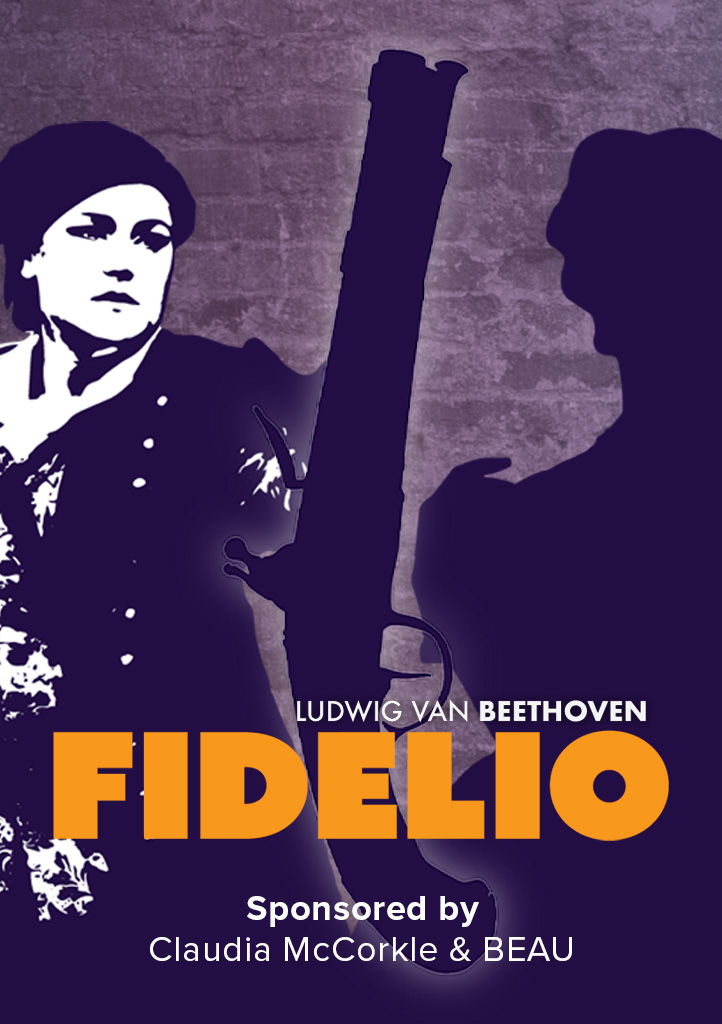The image is a dark, purplish-toned poster, possibly an advertisement or cover for a show or book, featuring a composite of computer-animated figures and graphical elements. Dominating the composition is a backdrop of a brick wall with some cement patches. On the left-hand side stands a woman in a black hat and a jacket, embellished with white buttons and a floral design. She also appears to wear a white scarf. On the right-hand side, there is a shadowy silhouette of another person, whose back is to the viewer, making it difficult to discern any distinct features or gender.

Centrally positioned in the image is an old-school, short-barreled gun, adding a dramatic focal point. Text overlays the scene: "Ludwig van Beethoven" is written in white, while "Fidelio” is prominently displayed in gold text. At the bottom of the poster, it reads "Sponsored by Claudia McCorkle & Beau” in white letters. This evocative and moody composition, with its rich details, suggests an intricate narrative or dramatic event possibly related to a concert or theatrical performance.